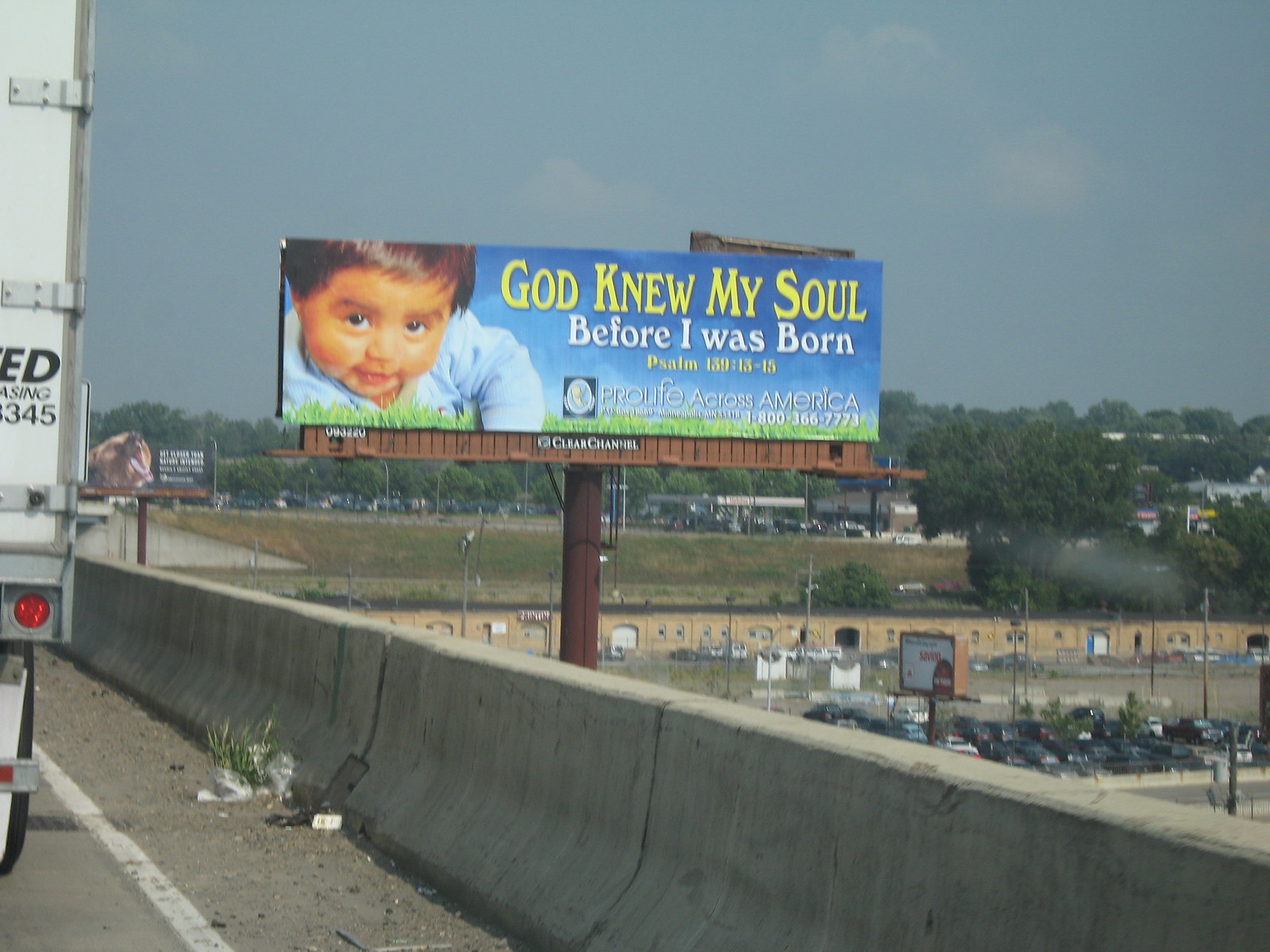This photograph captures a person crossing an overpass adorned with billboards. Prominently, one billboard features a child's image and advocates for pro-life, bearing the message: "God knew my soul before I was born" by Pro-Life Across America, sponsored by Clear Channel Billboards. Another indistinct sign is visible further in the background. Below the overpass, a parking lot stretches out, adjacent to a fenced-in area with a patch of dry ground. Behind this fenced area stands a gas station, with several trees dotting the landscape. A large semi-truck is seen driving along the left side of the image, adding a dynamic element to the scene.